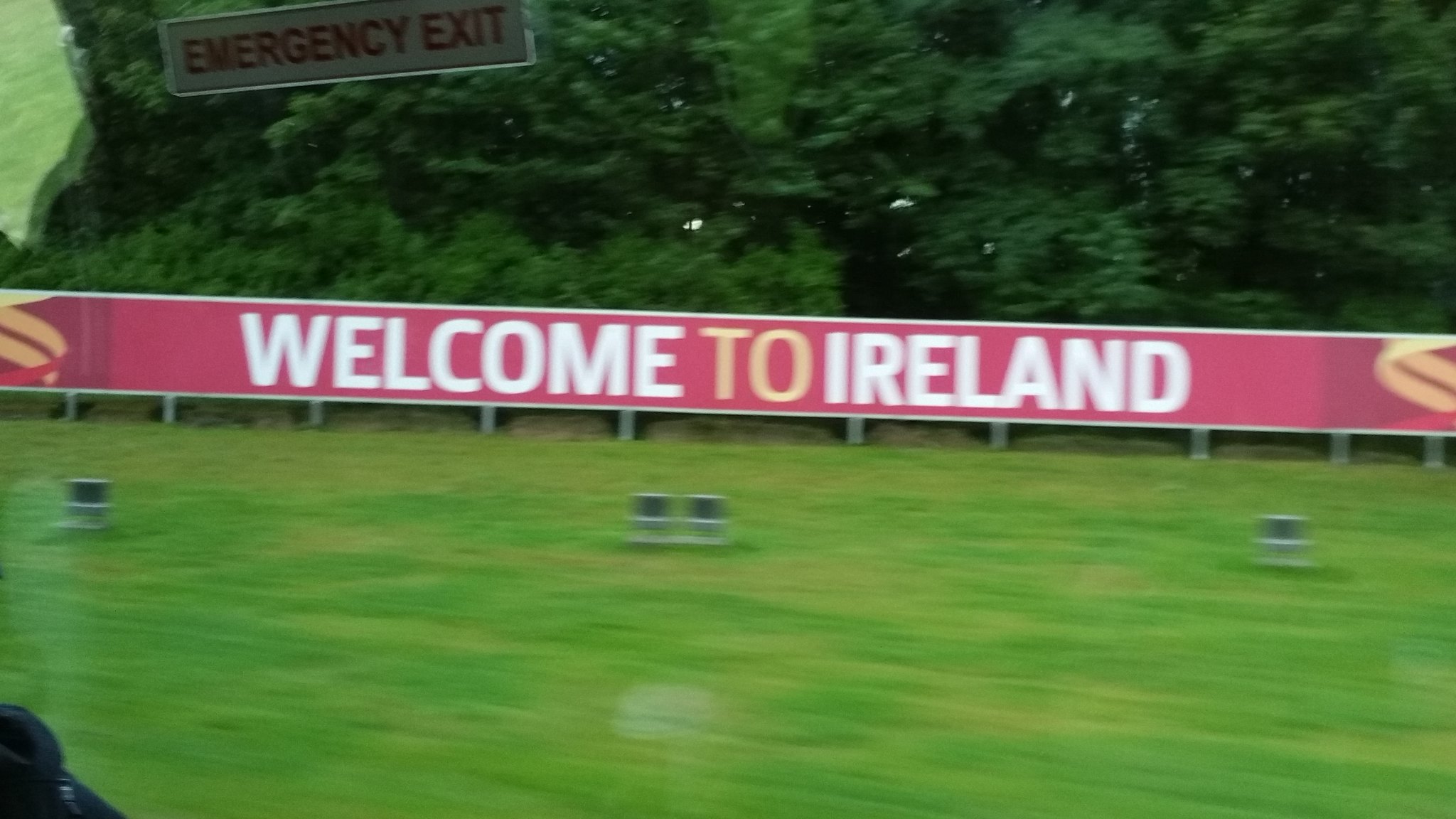This outdoor photo captures a vibrant scene centering on a long, thin billboard set against a lush natural backdrop. The prominent billboard features the word "WELCOME" in large, bold, white capital letters, followed by the word "TO" in striking yellow, and finally "IRELAND" in matching large, bold, white capital letters. Complementing the text, intricate yellow swirls embellish both the right and left sides of the billboard, harmonizing with the yellow of the word "TO." Surrounding the red billboard is a verdant landscape, with luxuriant green trees providing a scenic backdrop. In the foreground, a spacious grassy field extends towards the viewer, punctuated by a single metal post emerging from the grass, adding an element of industrial starkness to the idyllic setting. The overall composition balances the welcoming message of the billboard with the serene beauty of the natural environment.